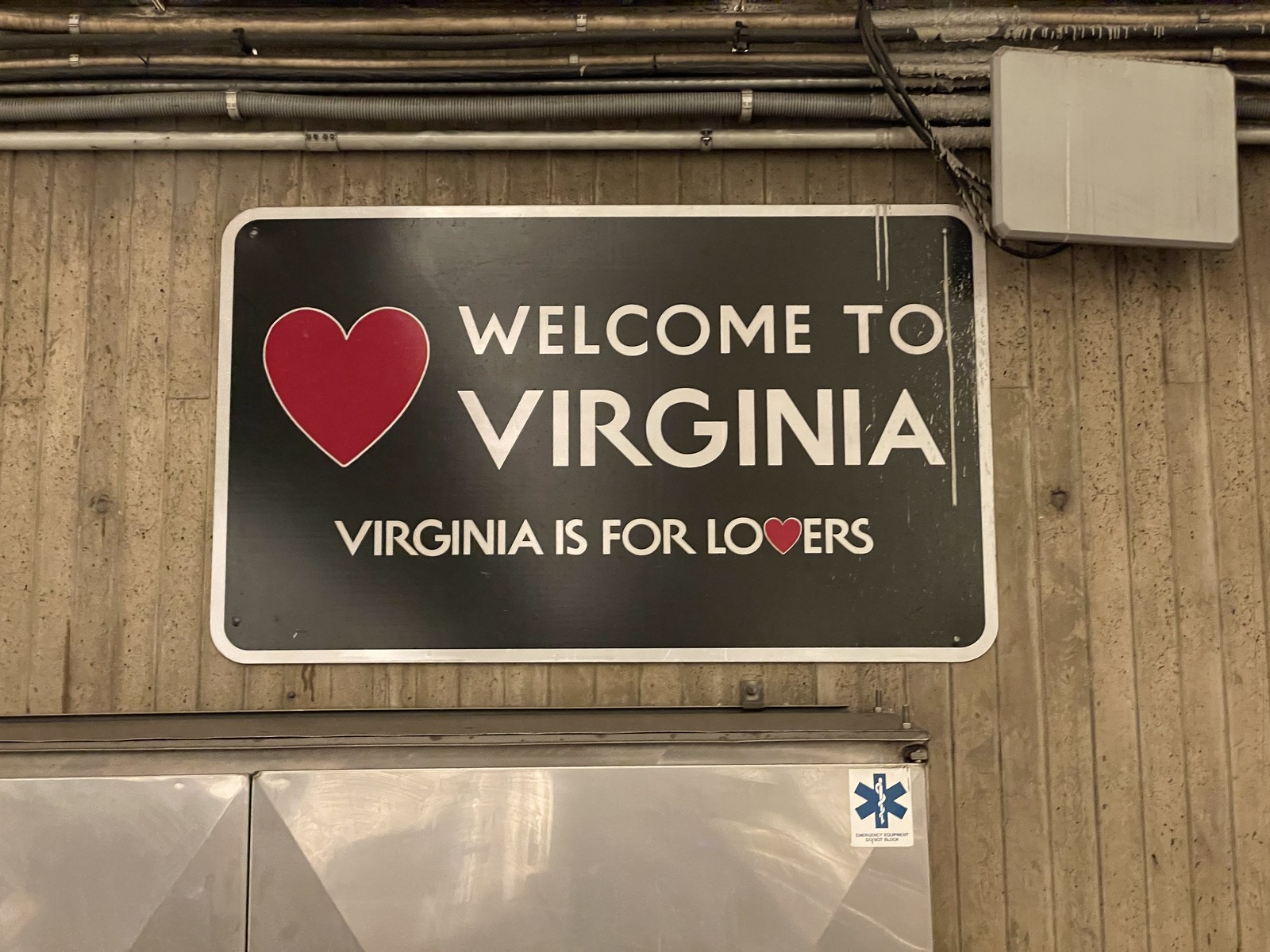The image depicts a rustic wooden wall made of vertically aligned, thin brown planks with natural wood markings. Centrally attached to the wall is a horizontally rectangular sign with a white border and black background, showcasing a red heart with a white border on the left. The sign reads "Welcome to Virginia," followed by "Virginia is for lovers," where the "V" is shaped as a red heart. Above the sign, near the ceiling, five long cables are stacked horizontally in colors silver, black, and dark brown. Toward the upper right, a gray, label-less box is situated below some pipes, with a black wire running from above the pipes down to the box. Lower left of the sign, there's a tan object with a metallic reflective surface, possibly a radiator. The setting evokes the image of a barn-like structure, adding a homely and welcoming feel to the scene.